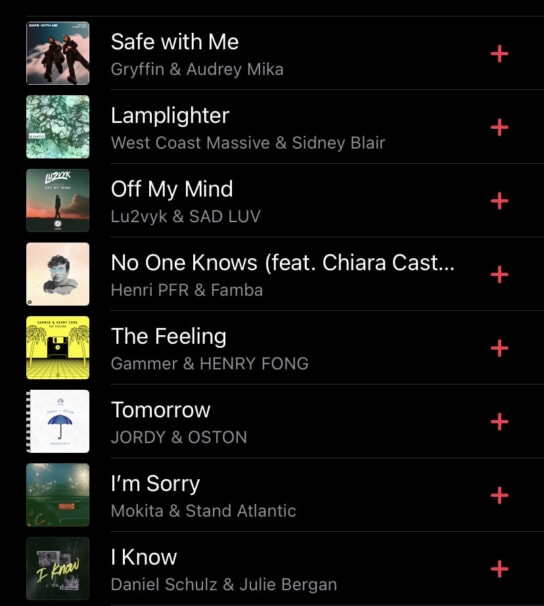In this rectangular image, we observe a screenshot displayed against a solid black background. This image showcases a list that appears to be songs and their respective artists. On the left side of each song title, there is a small square photo, likely representing album artwork or band images.

Starting from the top, the list includes:
1. **"Safe With Me"** by Griffin and Audrey Micah, presented in white text.
2. **"Lamp Later"** by West Coast Massive and Sydney Blair.
3. **"Off My Mind"** by Lou 2VYK and Sad Love.
4. **"No One Knows"** featuring Chiara Cast, Henry PFR, and Famba.
5. **"The Feeling"** by Gammer and Henry Fong.
6. **"Tomorrow"** by Jordy and Austin.

Each song title and artist name is distinctly separated, making the list clear and easy to read against the dark background. The square photos align perfectly with the song titles, adding visual interest to the otherwise text-heavy screenshot.